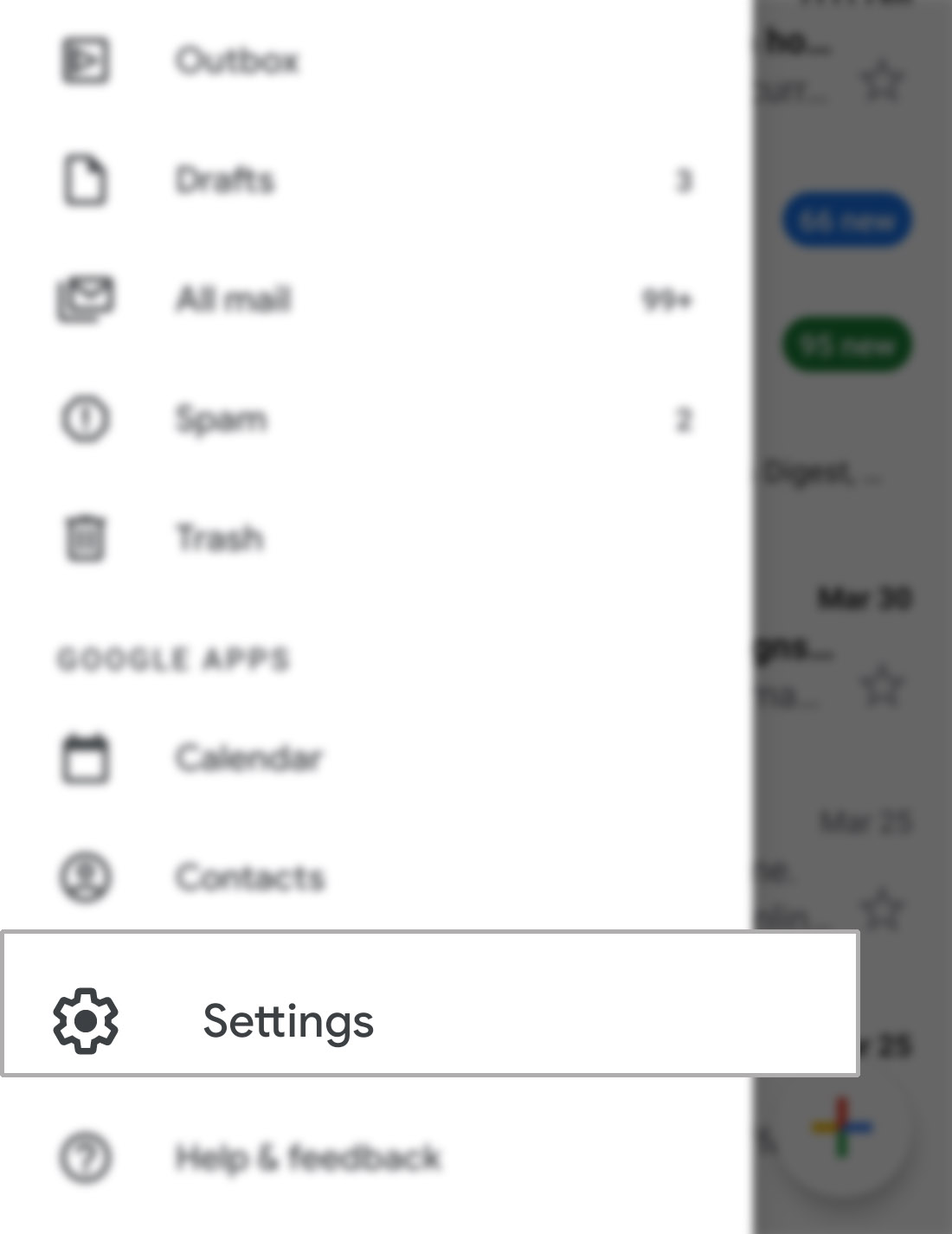A blurry image captured from a cell phone screen depicts a vertical menu on the left side, with "Settings" being the only clearly readable word, outlined in a gray rectangle. The vertical menu includes options such as Outbox, Drafts (3), All Mail (99+), Spam (2), Trash, Google Apps, Calendar, Contacts, Settings, and Help and Feedback. The far right side of the image faintly reveals part of the background. This image, taller than it is wide, contains no photographic elements, people, animals, birds, plants, flowers, trees, buildings, vehicles, or bodies of water.